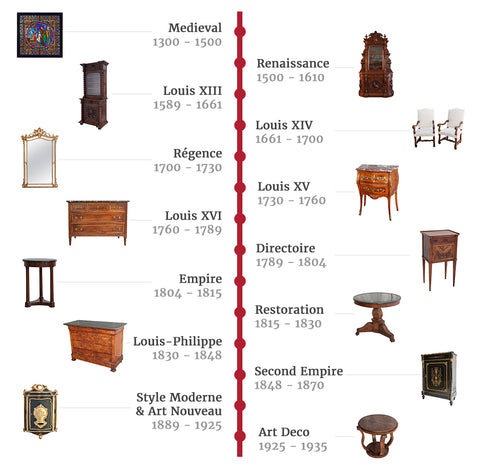The image showcases a detailed timeline of furniture styles spanning from the medieval era to the Art Deco period. A prominent vertical red line runs down the center against a white background, marking significant historical periods and their corresponding dates. The timeline starts with the medieval era (1300-1500), represented by an image of a stained glass window. Following this, the Renaissance period (1500-1610) is depicted with an ornate wooden dresser. Successive eras are highlighted with distinct pieces of furniture, indicating their stylistic evolution through time:

- Louis XIII (1589-1661)
- Louis XIV (1661-1700)
- The Regency period (1700-1730)
- Louis XV (1730-1760)
- Louis XVI (1760-1789)
- The Directoire period (1789-1804)
- The Empire period (1804-1815)
- The Restoration period (1815-1830)
- Louis Philippe (1830-1845)
- The Second Empire (1848-1870)

The timeline also features styles from the late 19th and early 20th centuries, including:
- Art Nouveau (1889-1925)
- Art Deco (1925-1935)

Various furniture pieces—ranging from tables and end tables to chairs, mirrors, and bureaus—extend outwards from the red line, each associated with its respective time period. This timeline vividly illustrates the progression and transformation of furniture design over more than six centuries.